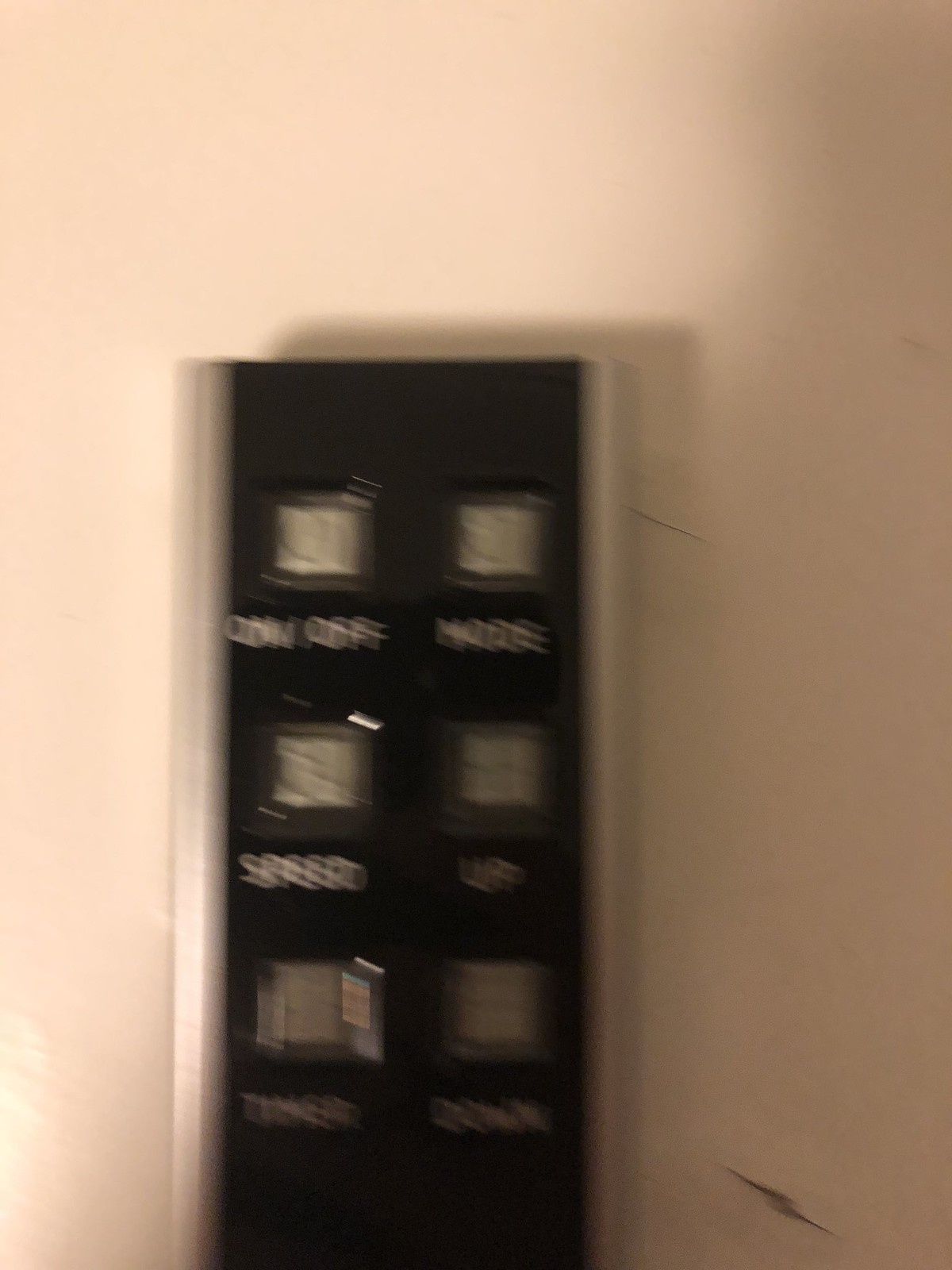This is a blurry, out-of-focus photograph of a black remote control. The image is taken against a light-colored background, possibly white or light pink, with some shadowing visible on the right side due to the low light. The remote control is vertically aligned slightly to the left of the photograph and extends beyond the lower edge of the image. It is primarily black plastic with thin silver strips on the left and right sides. The remote features six square buttons arranged in three rows of two. Each button has a corresponding white label in all caps beneath it. The top row includes buttons labeled ON-OFF and MODE. The second row has buttons labeled SPEED and UP, while the third row contains TIMER and DOWN. The overall blurry quality of the photograph makes the details hard to discern, but the general layout and purpose of the remote are clear.